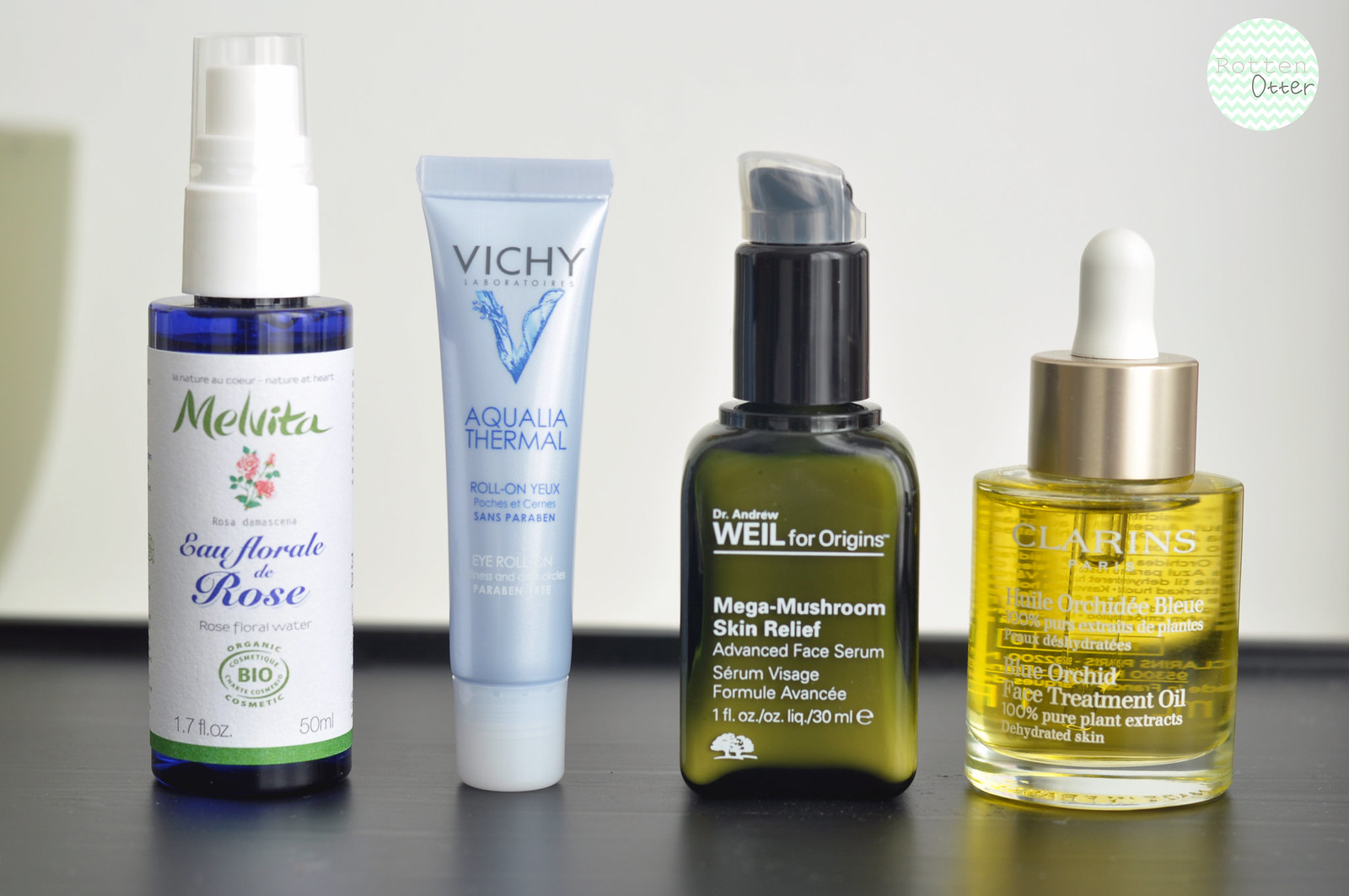This color photograph captures a still life of four beauty products elegantly arranged on a dark, polished surface, with a plain white wall as the backdrop. A watermark featuring a white circle with a green zigzag pattern and the text "Rotten Otter" is visible in the top right corner.

From left to right, the lineup of beauty items begins with a blue plastic bottle featuring a spray top protected by a clear plastic cap. The white label on the bottle, marked with green lettering, reads "Melvita" and includes a small illustration of pink flowers and green leaves. Additional text includes "Rosa Damascus, Eau Florale de Rose, Rose Floral Water, Organic Cosmetic," and a green circle labeled "BIO." Other label details include "Cosmetique Charte" and "1.7 fluid ounces, 50 milliliters."

Next is a shiny, bluish-gray tube with a white cap, standing upright. It is labeled "Vichy Laboratories" above a stylized 'V' resembling splashing water. The product name "Aqualia Thermal" is prominently displayed, along with "Roll-On Yeux, Poches et Cernes, Sans Paraben," and "Roll-On Puffiness and Dark Circles, paraben free."

Following the tube is a square green glass bottle topped with a black pump and protected by a clear plastic cap. The label reads "Dr. Andrew Weil for Origins, Mega-Mushroom Skin Relief, Advanced Face Serum, Formule Avancée, 1 fluid ounce / LIQ. / 30 mL." A small drawing of two white trees is positioned in the bottom left corner of the bottle.

The final item is a round glass bottle filled to the brim with a golden-colored liquid, capped with a shiny gold stopper. The label identifies the product as "Clarins, Blue Orchid Face Treatment Oil, 100% pure plant extracts, dehydrated skin."